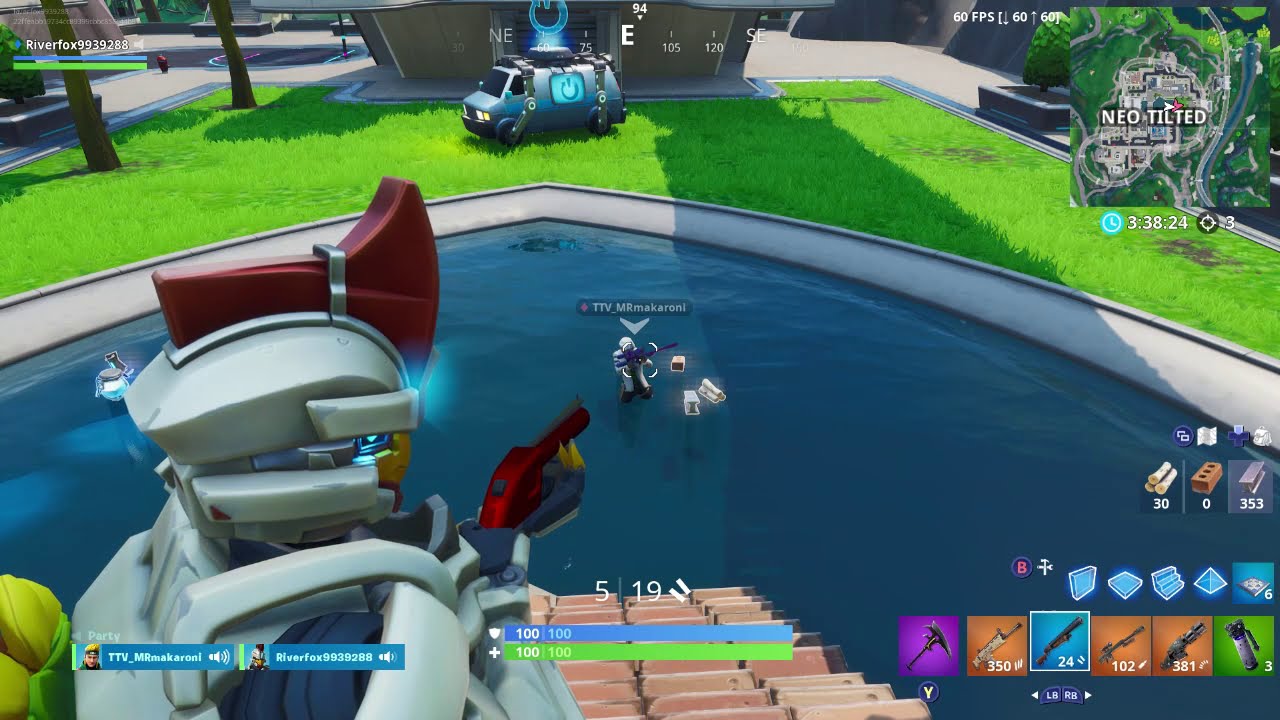This detailed screenshot from the video game Fortnite depicts a dynamic scene full of vibrant elements. In the bottom left corner, there's a character clad in white and red armor aiming a red gun at a character in the center of the image who is positioned in a pool of blue water. This scene is viewed from a third-person perspective. The water is surrounded by concrete sidewalks leading into a broad courtyard area. Bright neon green grass covers the top part of the image, along with some scattered trees, hedges, and a blue-gray van with paraphernalia on its roof, illustrating the outdoor environment within the game.

At the top right corner, the map named "Neo Tilted" is visible, indicating the in-game location. Along the bottom right of the image, an interface shows various weapon options colored purple, orange, and green, suggesting the player's inventory. The overall vivid color palette includes red, white, yellow, green, blue, purple, brown, and orange, adding to the lively and immersive nature of the game. This screenshot, which looks like it was taken from a console or computer, encapsulates the detailed and rich environment characteristic of Fortnite.